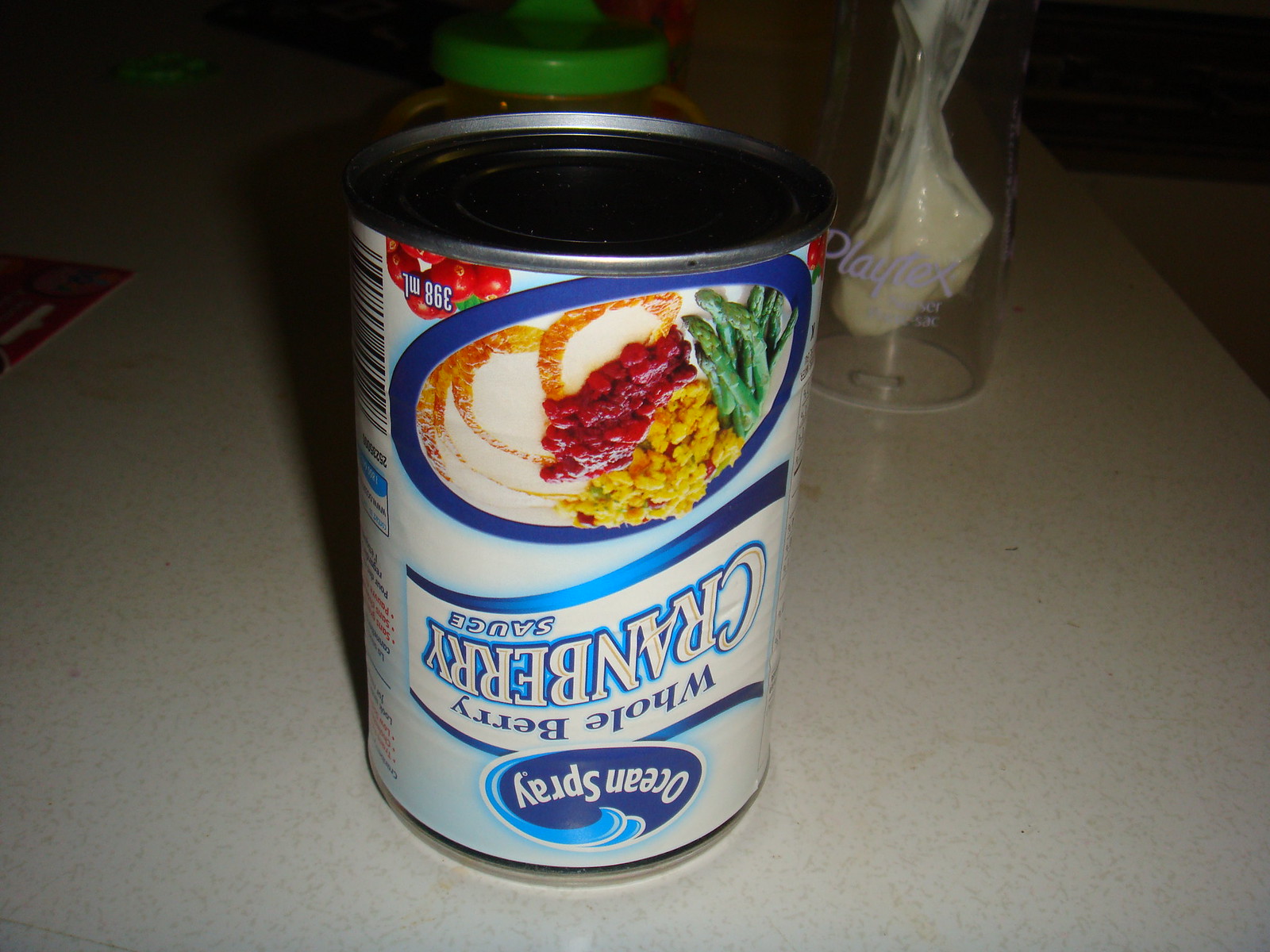A detailed, descriptive caption for the image:

"In this close-up photograph, likely taken with a point-and-shoot camera using flash, the main subject is an upside-down can of Ocean Spray Whole Berry Cranberry Sauce perched on a table. The flash illuminates the front of the can, causing a harsh shadow to be cast behind it. The can features vibrant, full-color packaging that prominently displays the text identifying the product. Below the text—appearing at the top of the inverted can in this image—is an appetizing illustration of a classic American Thanksgiving meal, complete with turkey, stuffing, and green beans, all meticulously arranged with cranberry sauce adorning the turkey. The rich colors and detailed depiction enhance the sense of a traditional holiday feast."